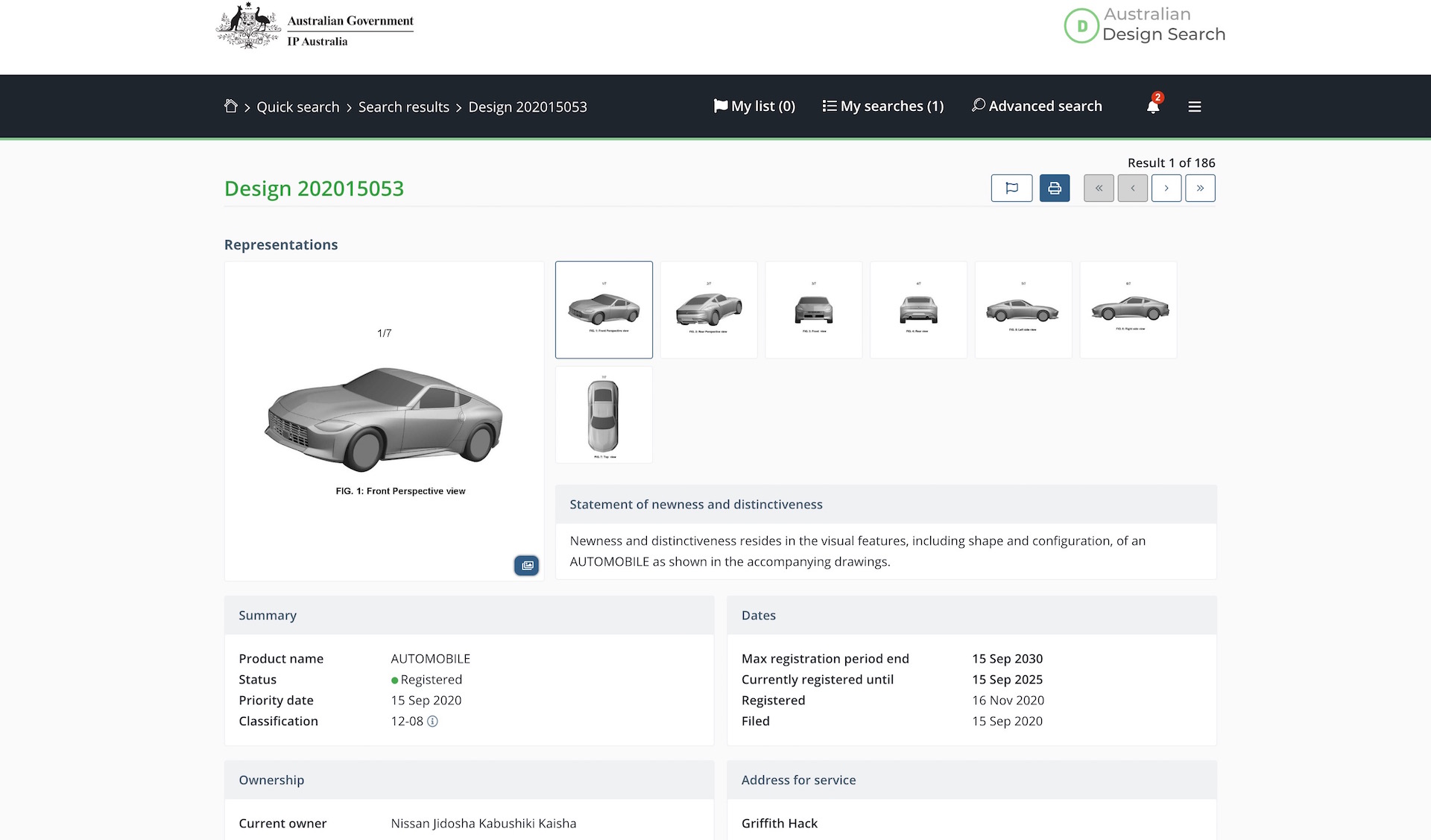The image depicts a car lookup page from the Australian Government IP Australia Design Search website. At the top of the page, there's a white banner displaying a slightly low-resolution logo of the Australian Government IP Australia. To the right of the logo, the text "Australian Design Search" is prominently featured, indicating that the page is related to design patents.

Below this, a black banner provides navigation options with labels such as "Quick Search," "Search Results," and "Design," along with an indication of the sequence number for this page. Additional options include "My List" with a count of zero, "My Search" showing one search, and "Advanced Search." There is also a bell icon with a red circle alert containing an unreadable number, suggesting pending notifications. The presence of a three-bar icon hints at a collapsible menu for additional options.

The main content area features a gray background with multiple white panels. The central panel prominently displays an image of a silver car, which appears to be a sports car, depicted from various angles in a sleek and aerodynamic design reminiscent of a computer-rendered model. Surrounding the primary image are several thumbnails arranged in a 6x2 grid, though the second row contains only a single thumbnail, offering multiple perspectives of the car.

Below the images, the page includes a summary of details related to the design patent, including key dates, the address for service, and other pertinent information about the intellectual property.

Overall, the page serves as a comprehensive interface for viewing and managing design patent information, complete with visual representations and detailed metadata.